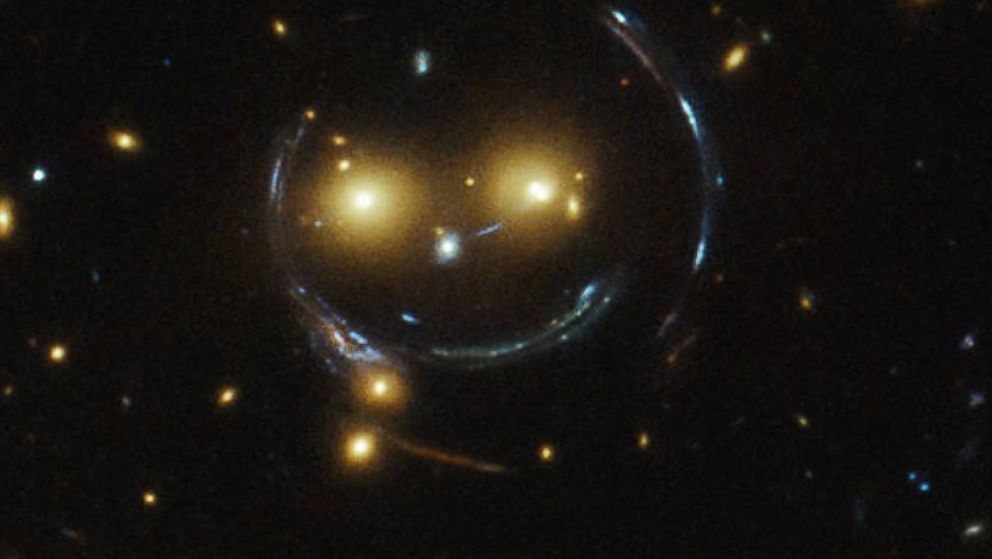The image depicts a captivating scene set against a dark black background scattered with small, white, and yellow dots resembling stars. Dominating the top middle of the frame is a striking formation that resembles a face. Two prominently bright, yellowish dots appear like eyes, and just below them is an intensely illuminated white dot, creating the impression of a nose. Encasing this facial feature is a translucent, bubble-like structure outlined with a light blue-white glow, reminiscent of a monocle or a shimmering fish shape. The bubble has a stretched, water droplet-like appearance, giving it an almost ethereal quality. Additionally, below the "face," there are more bright yellow dots, one of which is intersected by a faint brown line, akin to a stick. This mesmerizing and surreal assembly of lights and shapes creates an impression of an otherworldly gaze, staring into the vast, star-studded expanse.